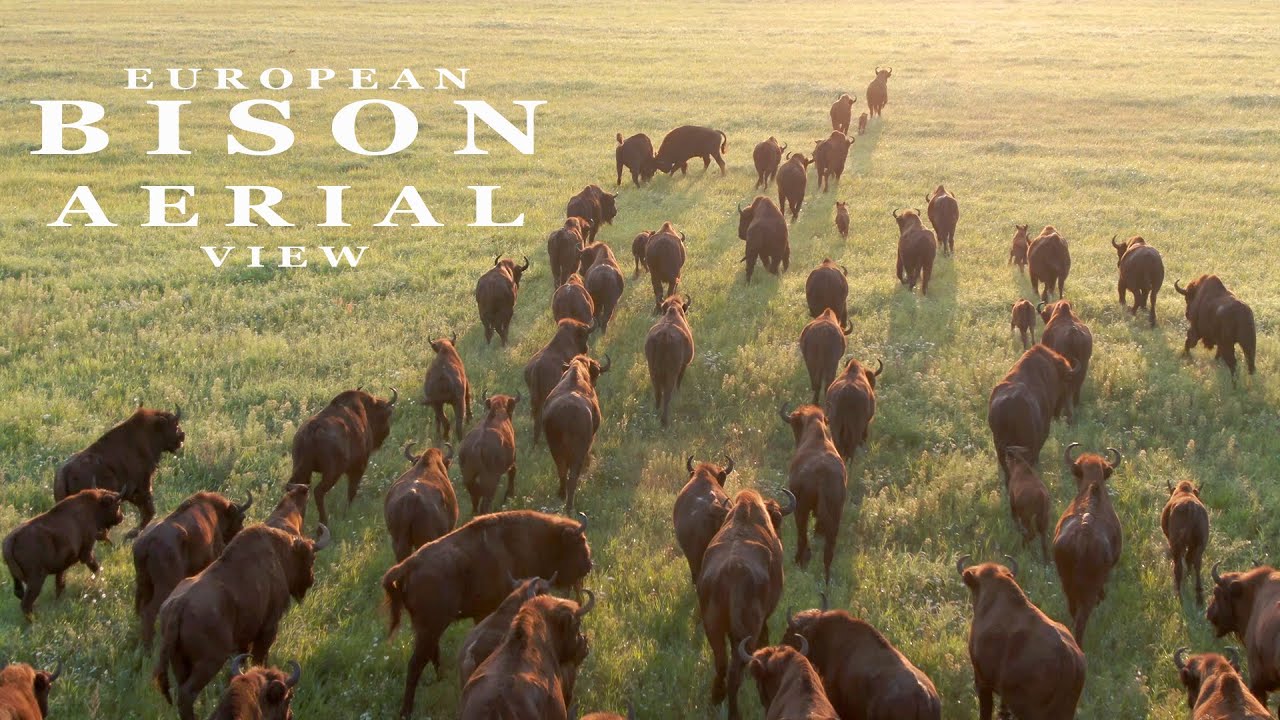This aerial drone photograph, in landscape orientation, provides a captivating view of a lush green meadow covered in grass and dotted with wildflowers. The scene is dominated by a large herd of European bison of varying sizes, some of which are calves. These dark brown creatures, identifiable by their short, curled horns and ridges of fur along their backs, move uniformly toward the top of the frame, creating a thick line across the landscape. The bison's movement casts long, dramatic shadows, suggesting the golden hour just after sunrise or shortly before sunset. The image is likely a cover page or thumbnail for a YouTube video or documentary, indicated by the title, “EUROPEAN BISON AERIAL VIEW,” displayed in spaced, capitalized white letters resembling Times New Roman font in the top left corner.